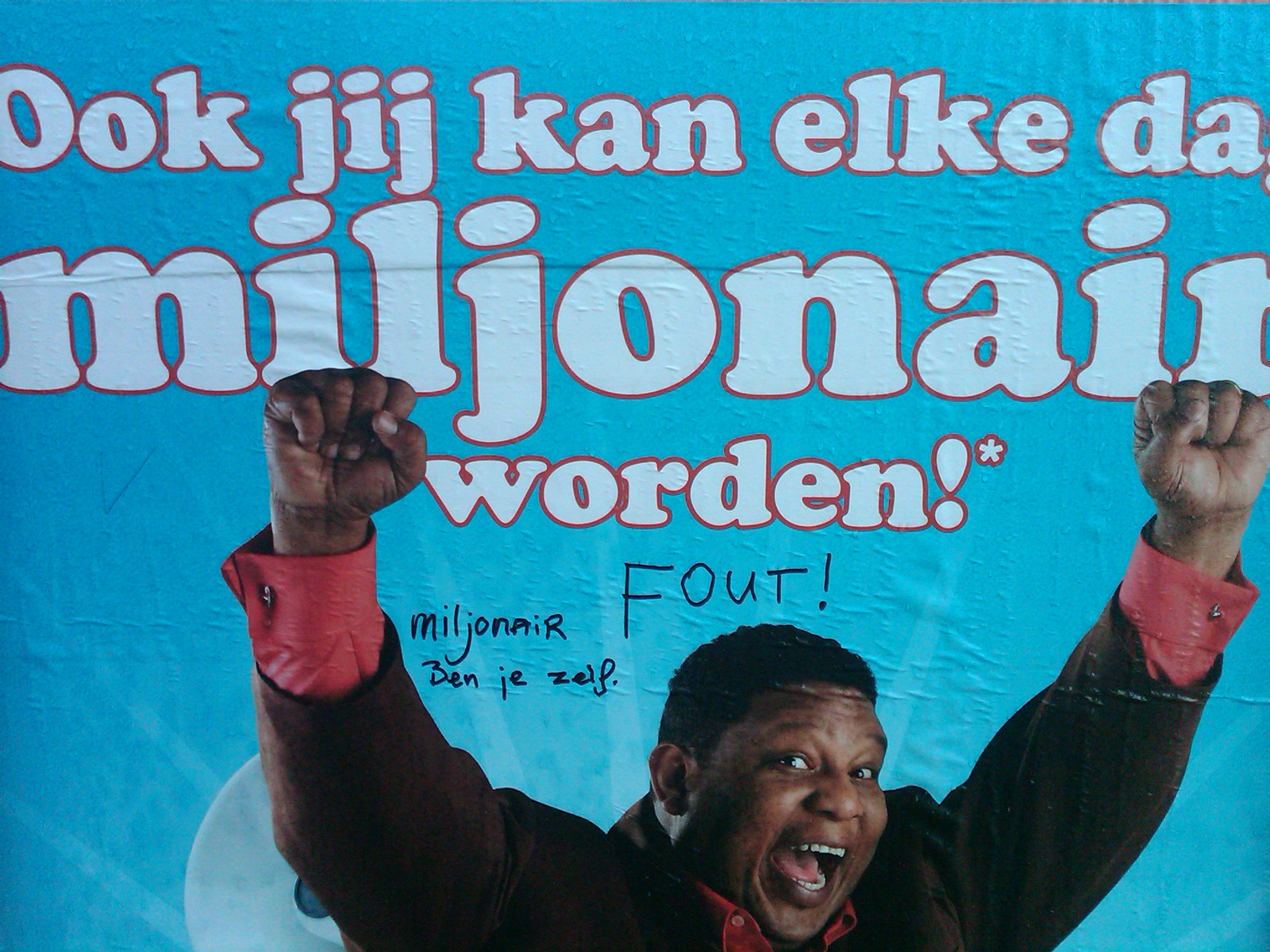This image features a vibrant advertisement painted on what appears to be a wall, adorned with a robin egg blue background. The centerpiece of the ad is a large, joyous black man depicted at the bottom, evidently ecstatic with his mouth wide open in a big smile, exposing his white teeth while his short black curly hair frames his animated expression. His arms are triumphantly raised, fists clenched, as if celebrating a significant victory. The man, who has dark brown skin and is larger in stature, wears a brown jacket with red sleeves peeking out towards his hands and a red shirt underneath. Above him, bold white letters outlined in red spell out what appears to be the foreign words "Ookjikon Elkida Miljonaire WORDEN" suggesting a connection to becoming a millionaire. The print medium shows noticeable ruffles and bubbles, giving it a texture of wear. Additionally, the word “FOUT!” is scribbled in black marker above his head, adding a layer of graffiti to the scene. The overall impression is that of elation and success, conveyed through vibrant colors and expressive imagery.